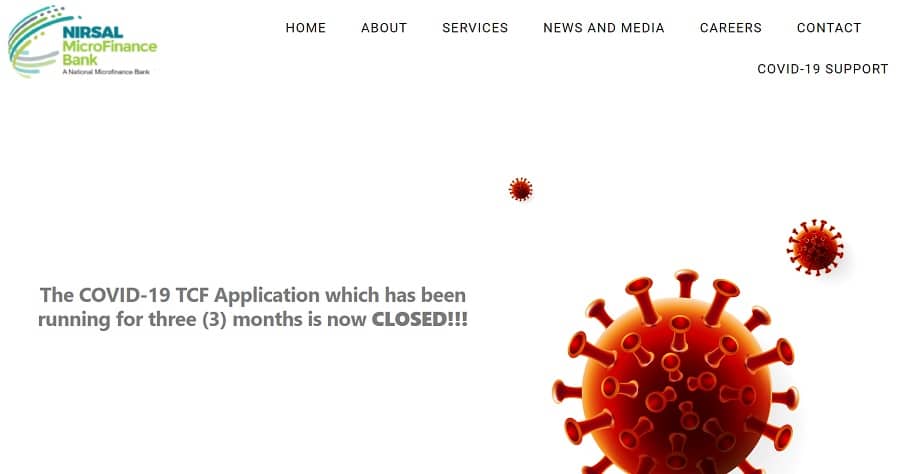The image appears to be a screenshot from a computer showing the webpage of the NIRSAL Microfinance Bank. In the upper left corner, the text "NIRSAL" is written in a teal color, followed by "Microfinance Bank" in green. Adjacent to this text, there is a graphic of curved lines in blue, gray, and teal.

To the right, the webpage features navigation headings: Home, About, Services, News and Media, Careers, and Contact, with an additional link under "Contact" labeled "COVID-19 Support."

At the bottom of the image, there is a section that combines text on the left and an image on the right. The text reads: "The COVID-19 TCF application, which has been running for three months, is now closed!!!" with "closed" highlighted in bold and followed by three exclamation marks.

The accompanying image on the right depicts a red circle with suction cup-like protrusions, likely representing the COVID-19 virus. Smaller and medium-sized illustrations of the virus are also present, one positioned to the upper left and the other to the upper right, all in a reddish-orange color.